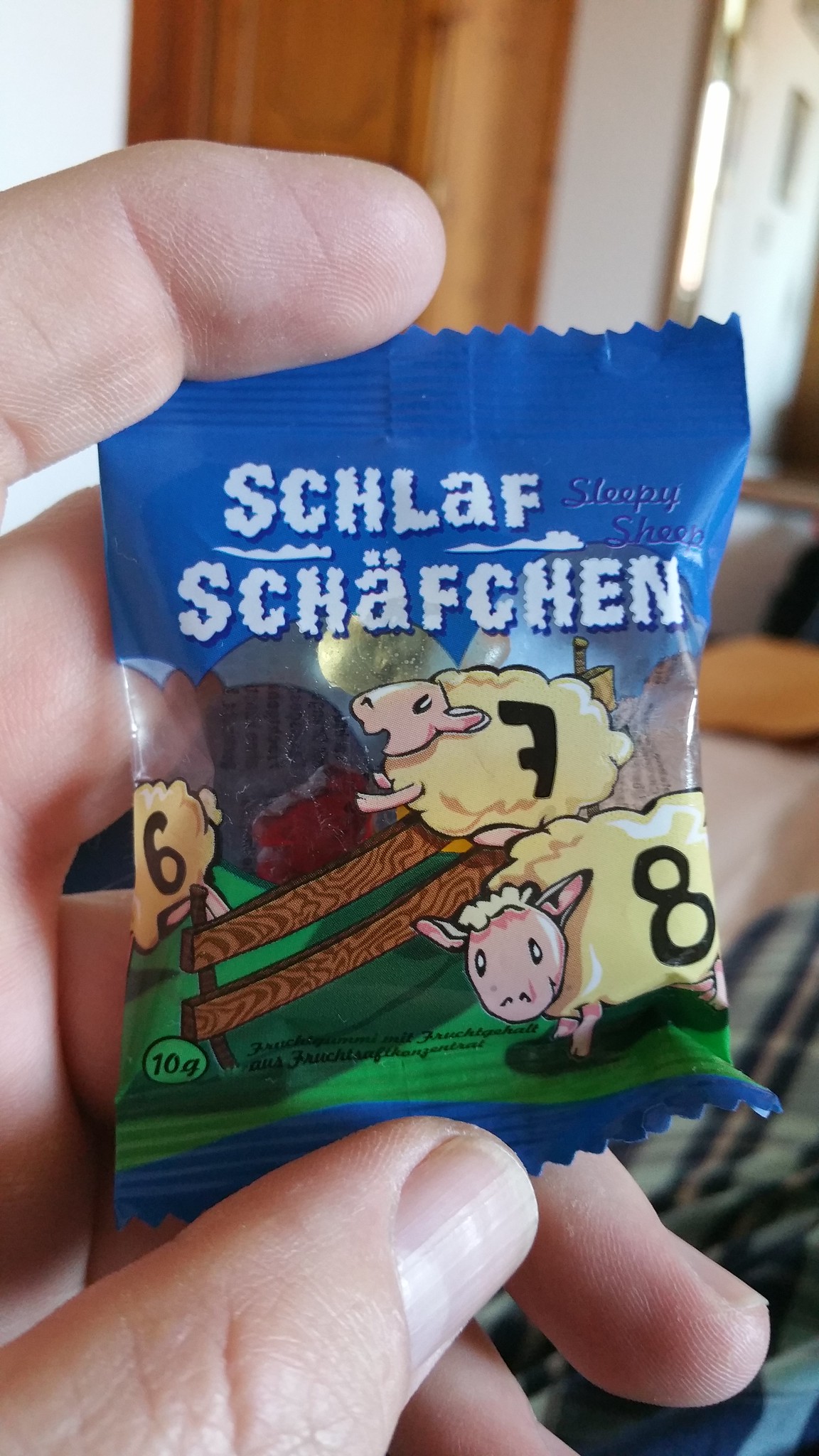The photograph captures a small plastic wrapper held by the fingertips of a person with white skin, set against a background that appears to be a standard room or possibly a hotel room. The wrapper is predominantly blue with light blue sections at the top and bottom, accented by a vibrant green background depicting a pastoral scene. On the front of the package, there are three cartoonish yellow sheep, each marked with the numbers 6, 7, and 8 in black. One sheep with the number 7 is depicted jumping over a wooden fence, reinforcing the theme of counting sheep to induce sleep. The packaging prominently features the words "Schlafschafchen," and below it, the English translation "sleepy sheep." A small icon indicates the weight as 10 grams. Within a clear section of the wrapper, you can discern two candies, one yellow and one red, likely suggesting the contents.